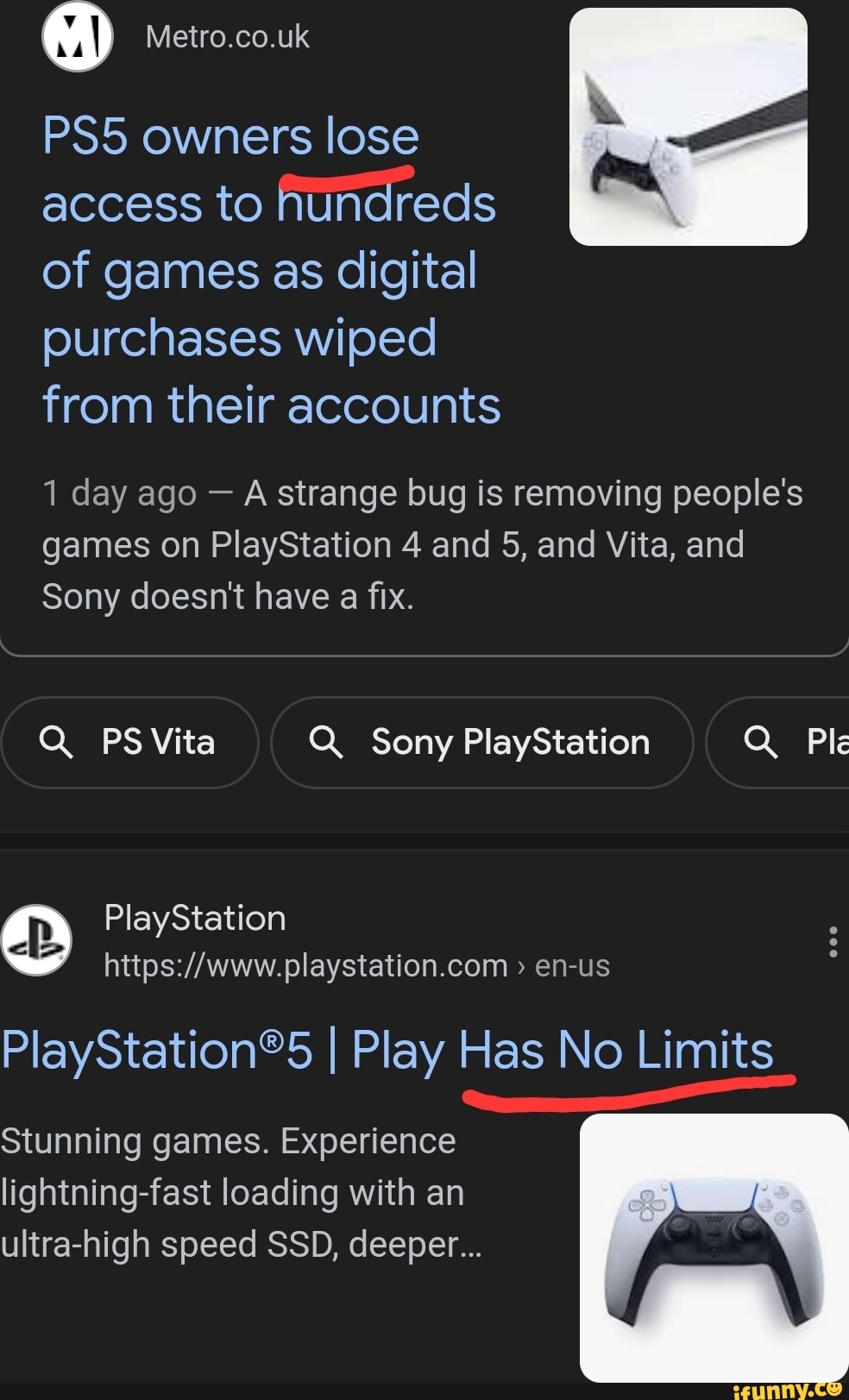In the image, a person is reading an article from the metro.co.uk on a dark background with blue text. The headline, prominently underlined in red, reads: "PS5 owners lose access to hundreds of games as digital purchases wiped from their accounts." Below it, a white-text subheading reveals, "One day ago a strange bug is removing people's games on PlayStation 4, 5, and Vita, and Sony doesn't have a fix." Following this, the article mentions key search terms such as "PS Vita," "Sony PlayStation," and "PlayStation," indicating the user's interest in the topic.

Adjacent to the main content, another section, marked with the PlayStation symbol, features a light blue text snippet: "PlayStation 5 - Play has no limits," with "has no limits" underlined in red. This is followed by a brief description extolling the console's capabilities: "stunning games, experience lightning-fast loading with an ultra high-speed SSD, deeper..." with the sentence trailing off in ellipses.

The peripheral visuals in the image include a picture of a PlayStation 5 controller next to the light blue text article and a PlayStation 5 console laying flat with a controller beside it accompanying the main article.